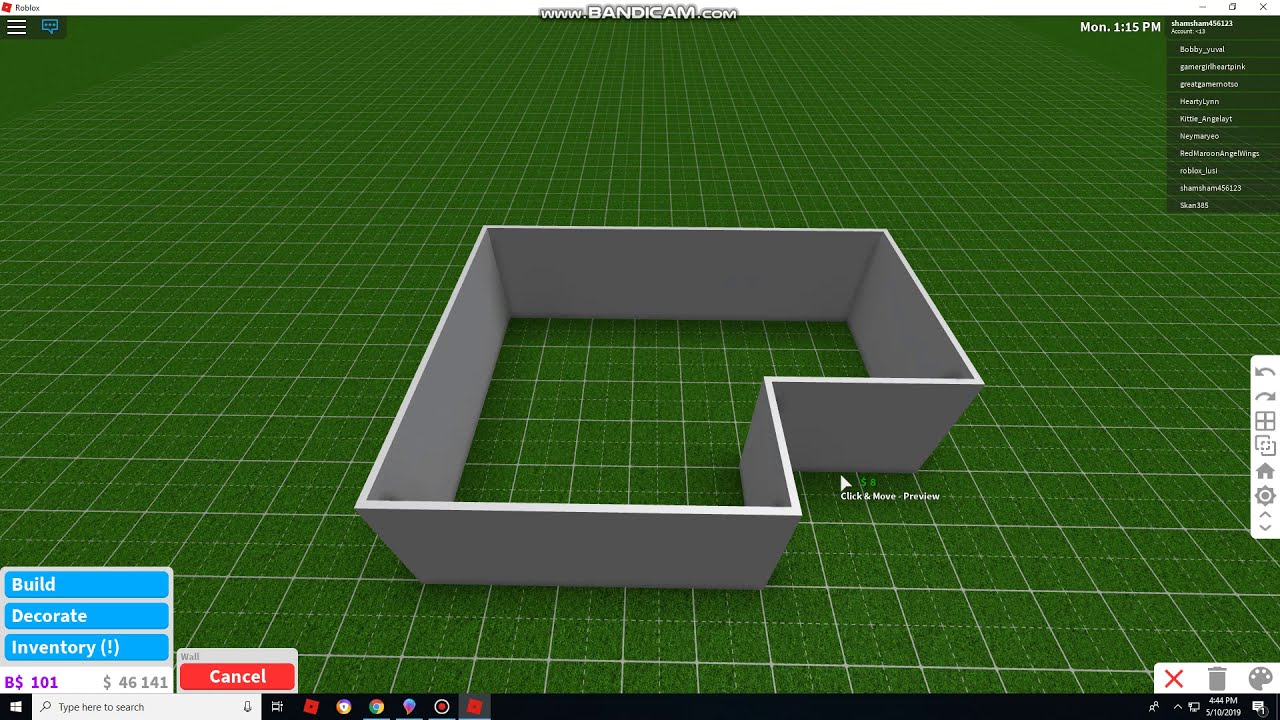The image is a detailed screenshot of the game Roblox in creation mode, specifically showcasing the build mode where a person appears to be designing a house. The main portion of the image reveals a 3D gray wall structure set atop a grid with a green, grass-like appearance. The grid is marked by intersecting white lines and dotted lines within the rectangles formed. The house's foundation comprises a rectangular body with an additional squared section extending downward from the left side, all featuring gray walls with bright white lining at the top.

In the bottom left corner of the image, there are three blue rectangles labeled "build," "decorate," and "inventory" in white font, alongside a display of in-game currency marked as "B$101" and "$46141." Additionally, a red rectangle labeled "cancel" is positioned to the right of these options. The bottom portion of the image includes a black strip resembling a computer's taskbar, featuring a search bar on the left, several icons to its right, and a timestamp in the bottom right corner.